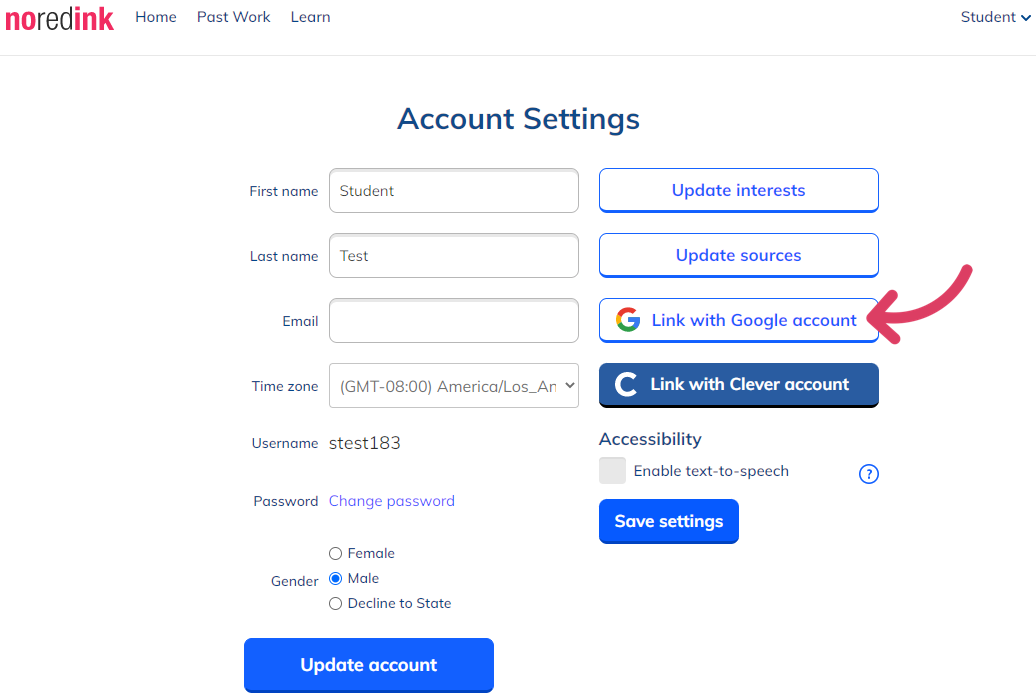Screenshot of the account settings page on the Nord Inc. website. At the top left corner is the Nord Inc. logo. Along the top navigation bar, from left to right, are buttons labeled "Home," "Password," and "Learn." On the far right of this navigation bar is a user icon with a dropdown menu. Underneath the navigation bar is a gray separator line, followed by the "Account Settings" section. 

In the "Account Settings" section, centered on the page, are various input fields and options. On the left side, it features labeled text input boxes for "First Name," "Last Name," and "Email." Each label is aligned with its respective input box directly to the right. Below the "Email" input box is a dropdown menu for selecting the "Time Zone." 

To the right of this dropdown menu, there is a button for linking a Google account, giving the user the option to integrate their Nord Inc. account with their existing Google account. This section allows users to update their personal information and account settings.